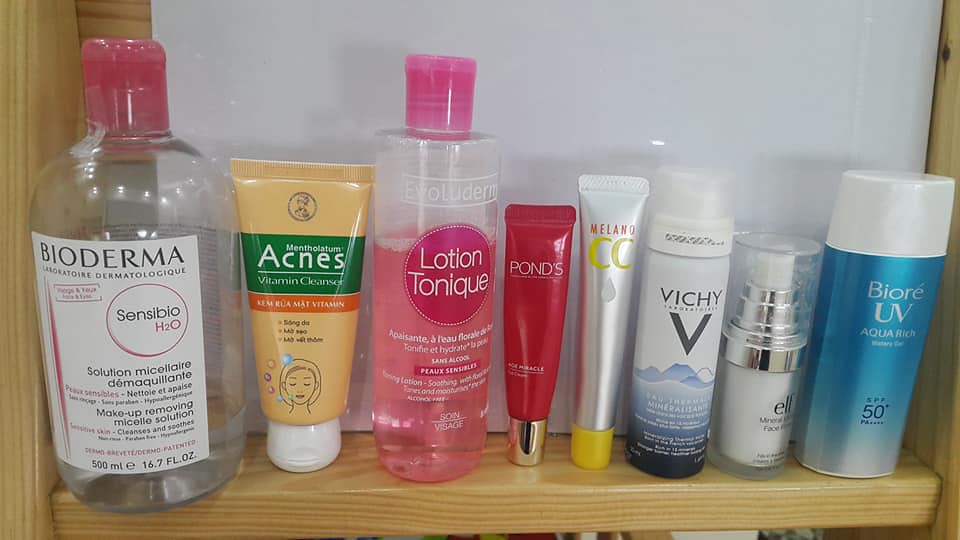This image depicts a bathroom shelf displaying an assortment of skincare products. The shelf itself is narrow, approximately 2.5 feet in length and 4-5 inches in depth. 

From left to right:
1. A large, clear bottle of Bioderma Sensible H2O Solution Micellar, identified by its pink lid.
2. A tube labeled ACNES with an animated female face, text in an ambiguous language, presumably Spanish.
3. Another large, clear bottle containing a pink liquid labeled Lotion Tonique, also featuring a pink lid.
4. A small, dark pink tube with a gold lid from the brand Ponds.
5. A thin, silver tube with a yellow lid, branded Wieland CC.
6. A larger canister labeled Veachie with a prominent 'V' and wave designs at the bottom; the top part is white.
7. Another container showing partial letters "EL," possibly indicating the brand ELF, with a pump dispenser on top and likely a face lotion.
8. Finally, a blue can of Biore UV Aqua with "50" towards the bottom, topped with a white lid.